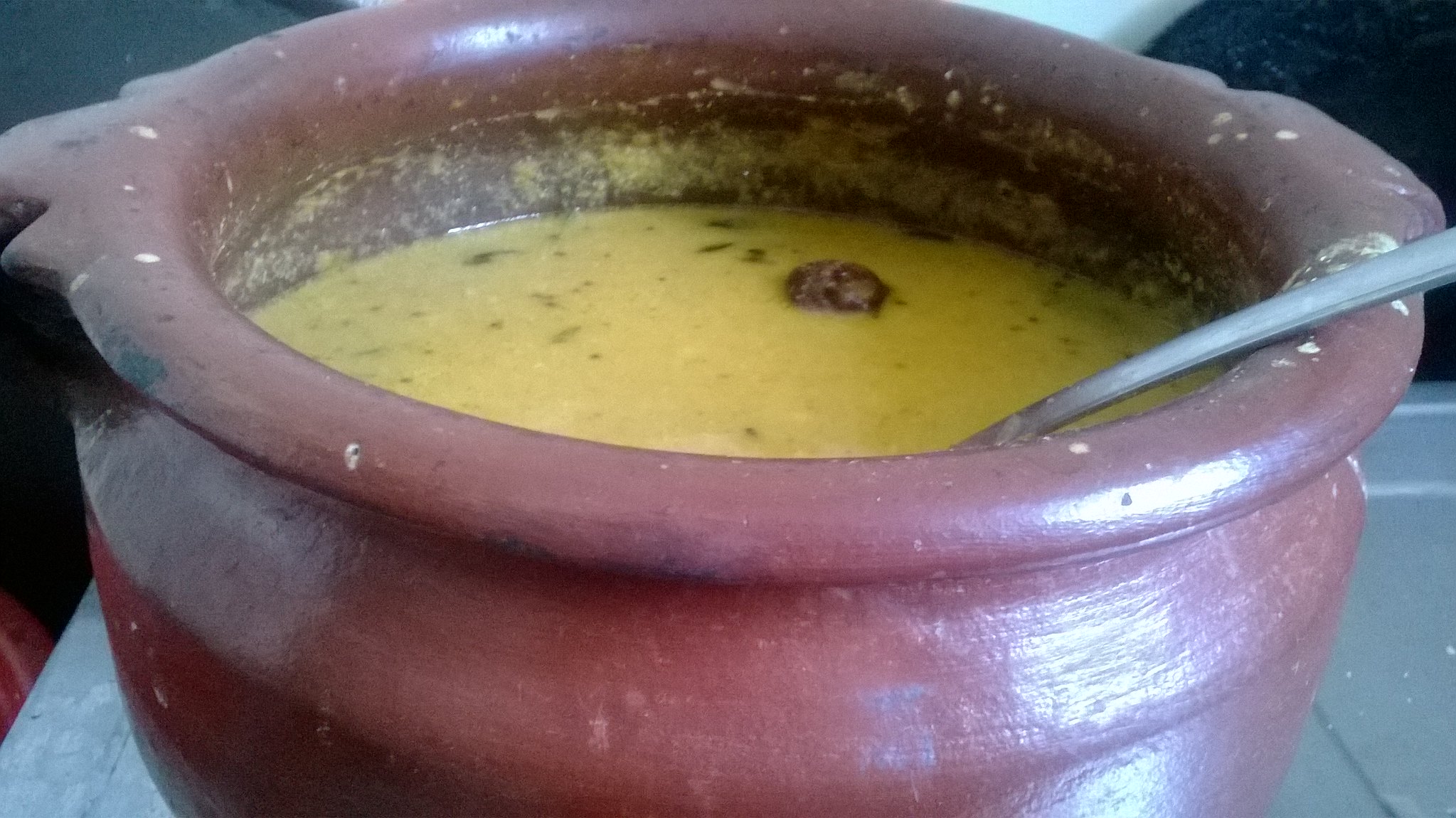The photograph shows a large, rustic clay pot with a wide lip and handle-like protrusions, sitting on a grayish-blue tabletop. The pot is predominantly a deep red or burgundy color with chipped areas revealing spots of white, hinting at age or wear. Inside the pot is a creamy yellow soup, speckled with green herbs, and floating in it are chunks of what appear to be red or brown vegetables or meatballs. A silver spoon is placed in the soup, suggesting it might soon be eaten. The setting appears to be indoors, with a dark and somewhat indistinct background, and a glimpse of a red cloth below the table in the lower left corner.